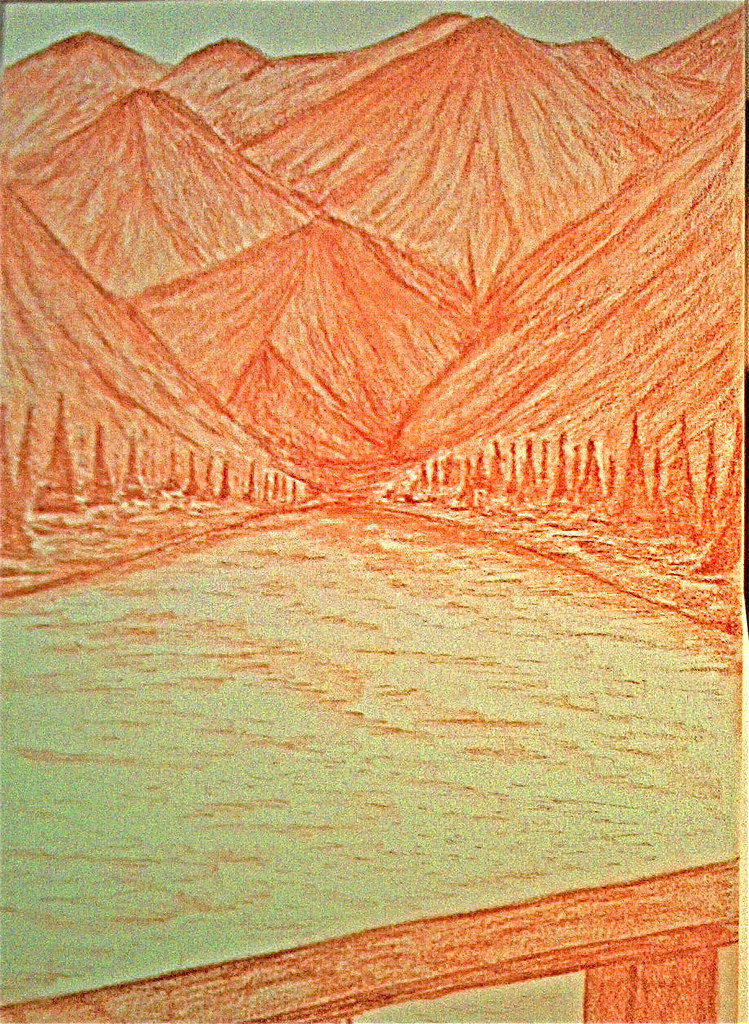The image is a detailed crayon or colored pencil drawing of a vibrant river valley framed by a majestic mountain range, rendered predominantly in shades of blue and reddish-orange. The background features a dramatic skyline in a bluish-green hue, accentuating the towering, multi-layered peaks of the mountains, which rise to various heights and descend toward the center, reminiscent of a box canyon. Orange-hued tree lines flank both sides of the scene, enhancing the autumnal atmosphere. The valley itself houses a flowing river, visually tapering from a wide foreground to a narrow end near the rocky mountain base, with intricate shading that simulates the shimmering motion of water. In the foreground, a wooden bridge rail can be seen, suggesting the viewer's vantage point is from a bridge, offering a panoramic view of the picturesque, expansive river valley.